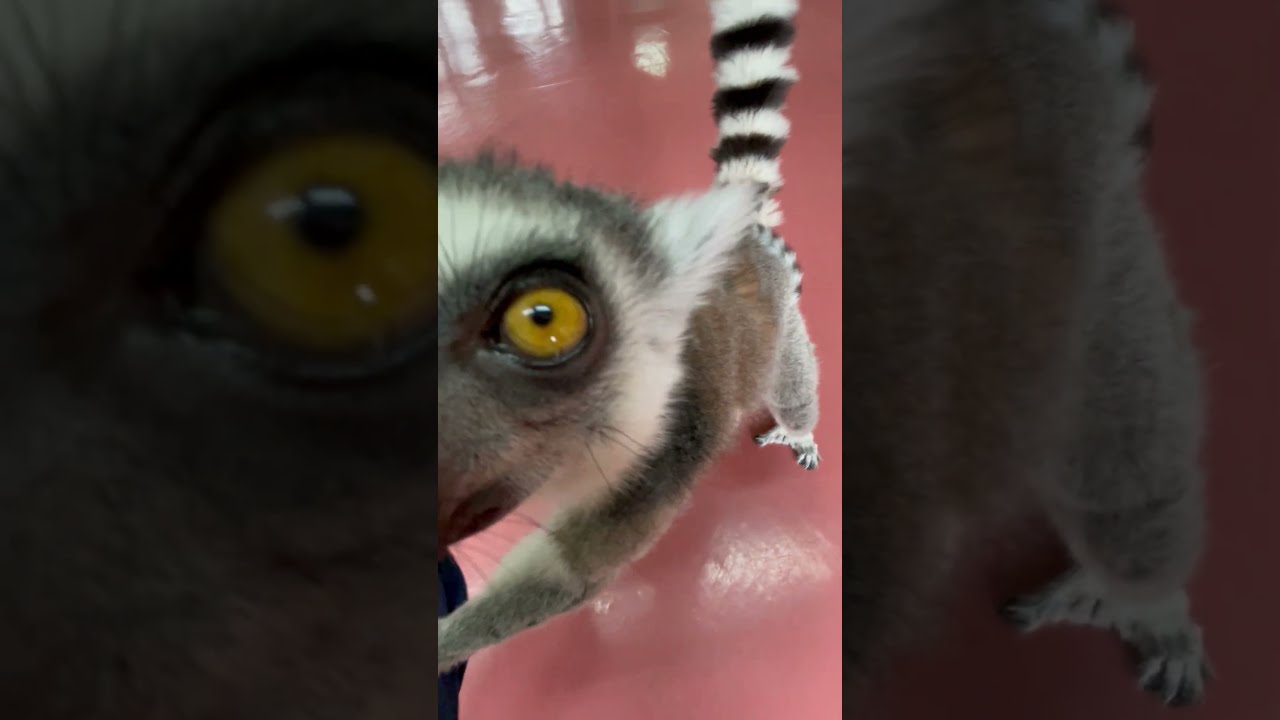The image depicts a close-up view of a lemur positioned centrally on a glossy, salmon-red tile floor, with light reflections accentuating the surface. The lemur's full body occupies the narrow, vertical rectangular center of the photo. Its striking golden-yellow left eye, with a black pupil, is prominently visible and appears to be looking up, possibly at a person or object of interest. The lemur's fur is a mix of gray, brown, and white, while its tail exhibits distinct black and white horizontal stripes. On both sides of the central image are darker, blurred close-ups: the one on the left focuses on the lemur's left eye, and the one on the right captures the back end of the lemur, including its tiny feet.